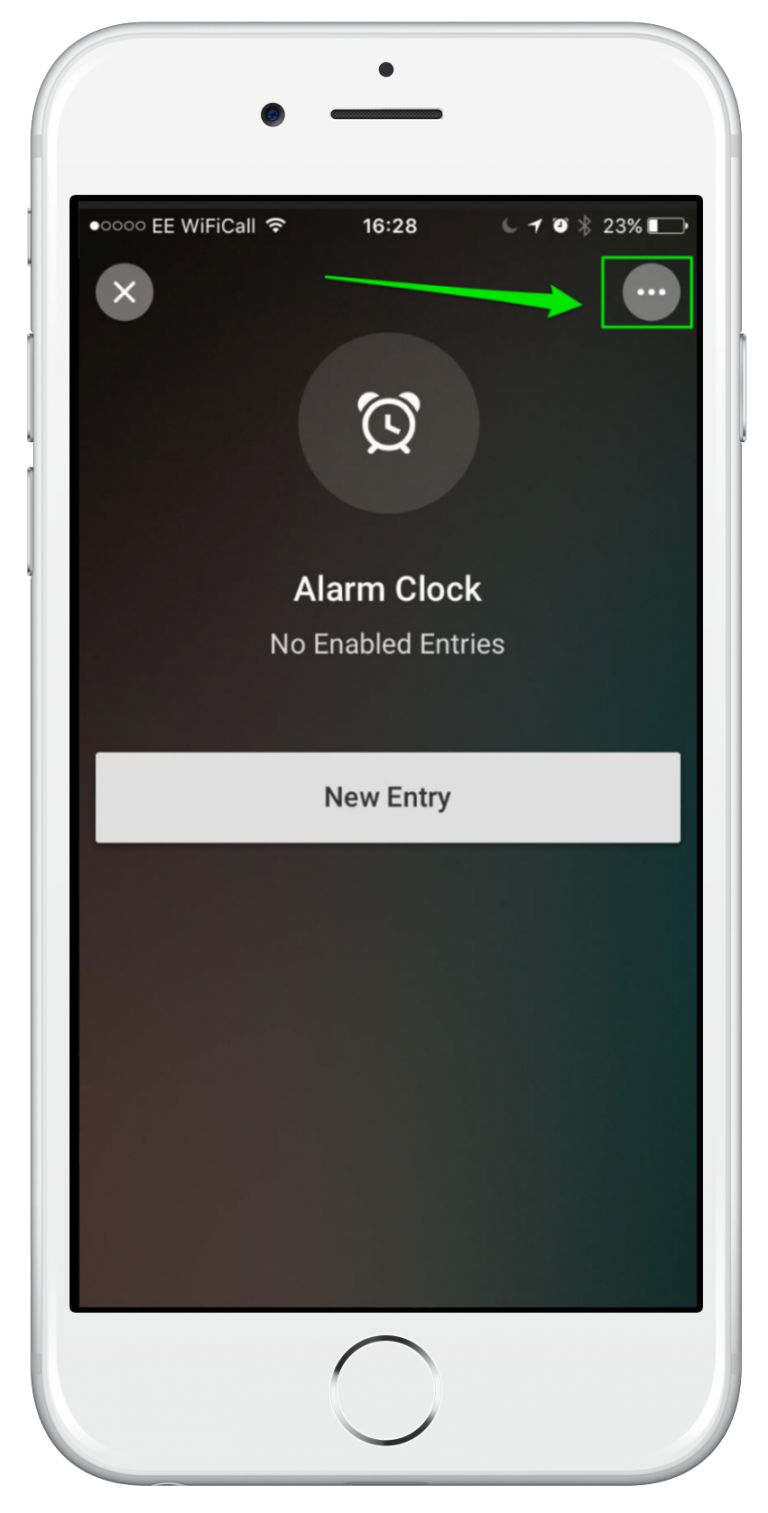The image depicts a silver iPhone displaying the alarm clock setup screen. The device's battery life is at 23%, as shown in the top right corner. The screen time reads 16:28, and the strong Wi-Fi connection icon is also visible. The main screen background appears black, featuring a large, black-gray circle in the center with a white alarm clock icon. Below this, it states "No enabled entries."

Within the black area, there is a white box containing the text "New entry." On the upper left side of the screen, there is a small gray box with an "X" inside. Additionally, a green box with three white dots is displayed, connected to the Wi-Fi icon by a green arrow—though its purpose is unclear. The overall design of the phone includes a silver exterior and a white interior.